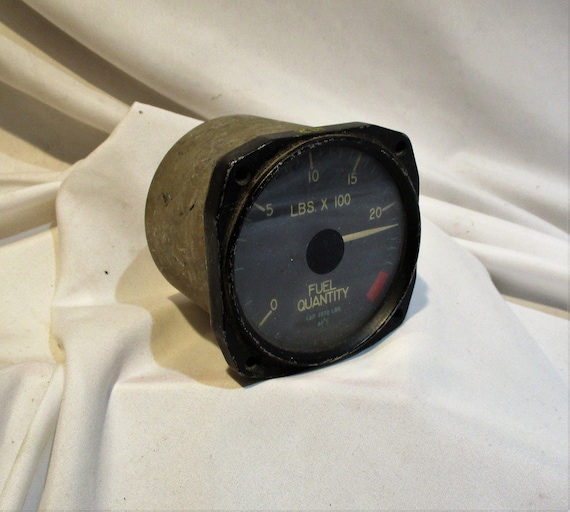This image showcases a cylindrical gauge, likely from a vehicle, placed against a neatly draped white cloth backdrop. The gauge features a black faceplate on top, with a circular glass front bordered by black edges. Inside, there is a dial resembling a speedometer or fuel gauge, marked with numbers from 0 to 20 in white. The gauge includes a red zone beyond the 20 mark, indicating a critical level. The white arm, or needle, in the center of the dial points to these numbers to show measurements. Across the top of the dial, it is labeled "pounds x 100," and beneath the needle, it reads "fuel quantity," indicating it measures fuel levels. The background drape appears to be used as a backdrop for the photograph, highlighting the cylindrical, metallic structure extending from the back of the gauge.